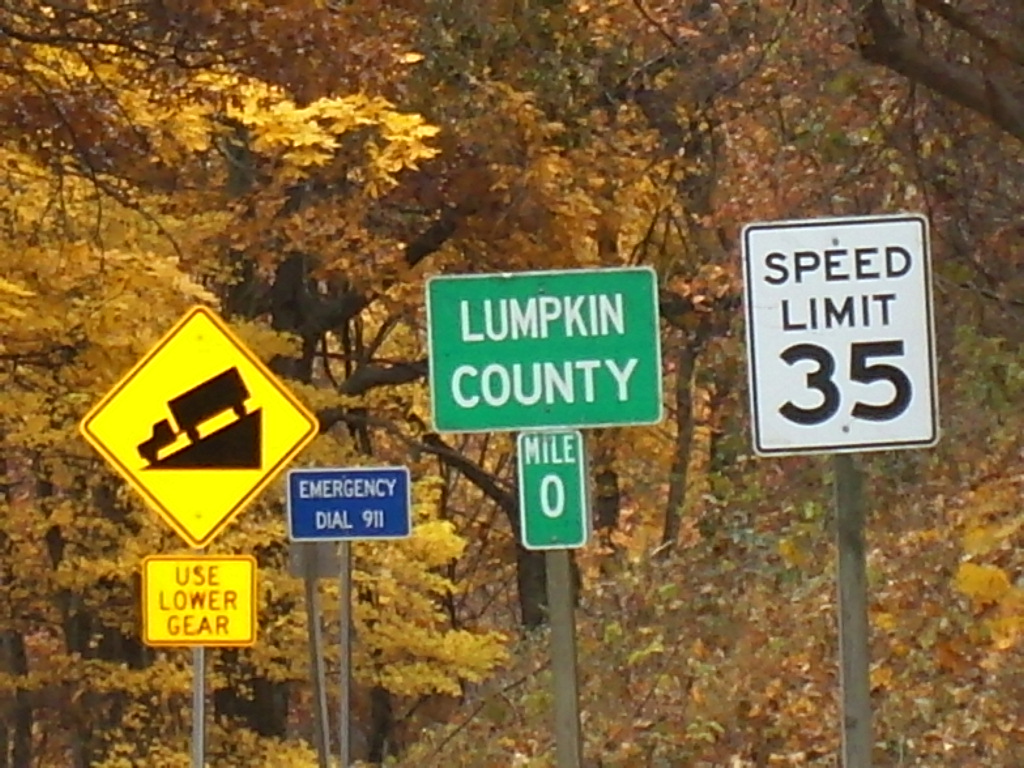The photograph displays a cluster of road signs against a backdrop of lush fall foliage dominated by vibrant yellow and gold tones. The image, slightly wider than it is tall by about 20%, features prominent and varied signage on what appears to be the side of a road. Starting from the right, there’s a vertical speed limit sign with a white background, black border, and bold black lettering that states “Speed Limit 35.” Adjacent to it is a green county sign with "Lumpkin County" in white text, and directly below it, another green sign indicates “Mile 0.” Further left, a blue sign with white text reads “Emergency Dial 911.” To the far left, there is a cautionary yellow diamond-shaped sign depicting a truck descending a steep hill, beneath which is a rectangular sign in the same yellow, instructing truckers to “Use Low Gear.” The signs are affixed to wooden or metal posts and stand out distinctly against the canopy of mostly yellow and some orange leaves with minimal visibility of the tree trunks, indicating a higher vantage point for the foliage.